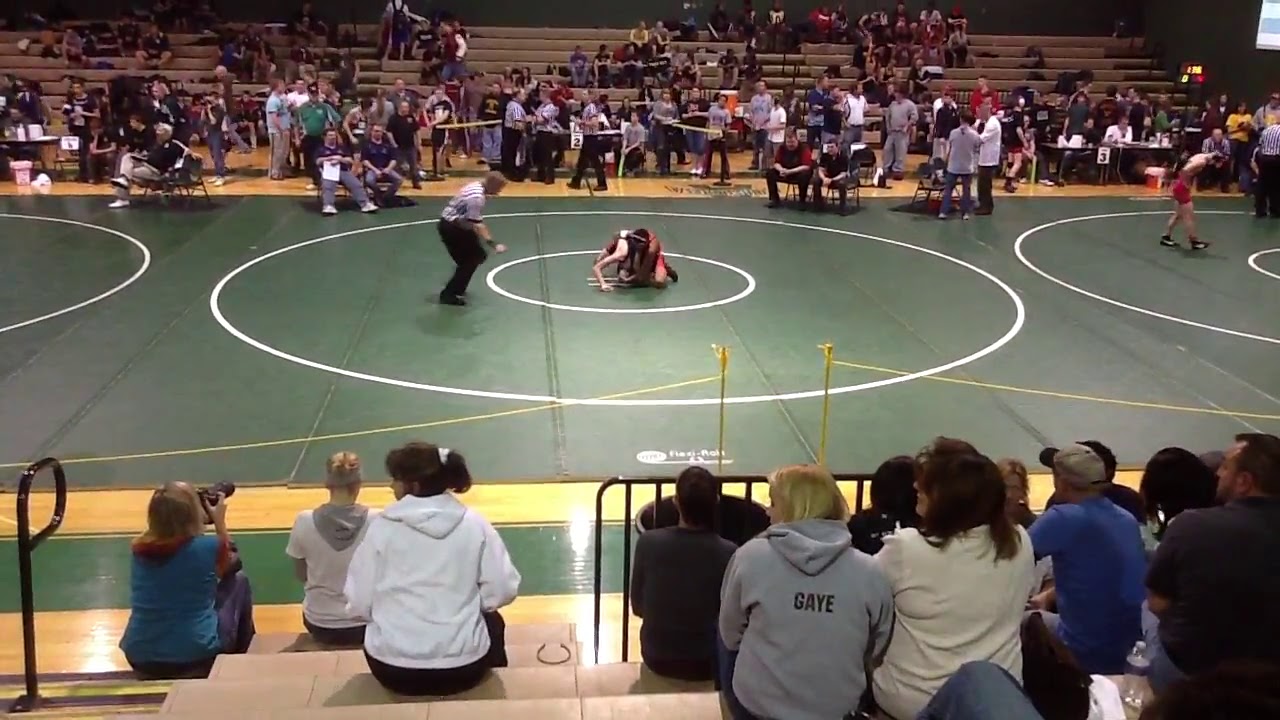The image captures an indoor wrestling match taking place in a gymnasium or stadium. The central focal point is a large green mat adorned with two concentric white circles. In the innermost circle, two young wrestlers are engaged in a match; one is dressed in black and the other in red. Both athletes are on their hands and knees, grappling intensely. To the left of the wrestlers, a referee dressed in a black and white striped shirt and black pants is squatting slightly, closely monitoring the match with his arm extended toward the ground.

Surrounding the mat is a glossy wooden floor, beyond which spectators fill the bleachers on both sides. The bleachers are bustling with people standing, sitting, and chatting, some with cameras, including a woman in a blue shirt and jeans with a long-lens camera capturing the action. In the foreground of the image, only the backs of seated spectators are visible, including a notable figure in a gray t-shirt with the name "Gay" on it.

In addition to the main match, groups of people are seated in chairs around the edge of the mat, and a table marked with the number three, likely signifying judges or officials, is visible on the right. Near this table, another wrestler stands prepared, hinting at an adjacent ongoing match. The image vividly encapsulates the dynamic and energetic atmosphere of a live wrestling event, where the action on the mat is mirrored by the engagement of the spectators.